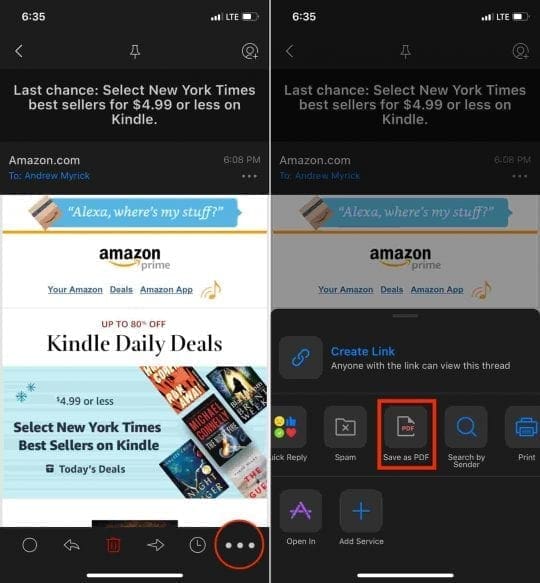Two side-by-side images captured from a smartphone screen display Amazon promotions and menus. Both images are timestamped at 6:08 PM and addressed to Andrew Myrick. At the top of each image, the words "Last Chance: Select New York Times Best Sellers for $4.99 or less on Kindle" are prominently displayed beneath the clock showing 6:35. 

In the image on the left, an Amazon page is shown with a banner advertising "Up to 80% off Kindle Daily Deals." Below this, on a light blue background, five book covers are featured along with the text "$4.99 or less: Select New York Times Best Sellers on Kindle Today's Deals."

In the image on the right, the Amazon Kindle page displays a different interface, highlighting several menu options. The option in the middle, which is enclosed in a red square, features a file icon labeled "PDF" and the text "Save As PDF" at the bottom.